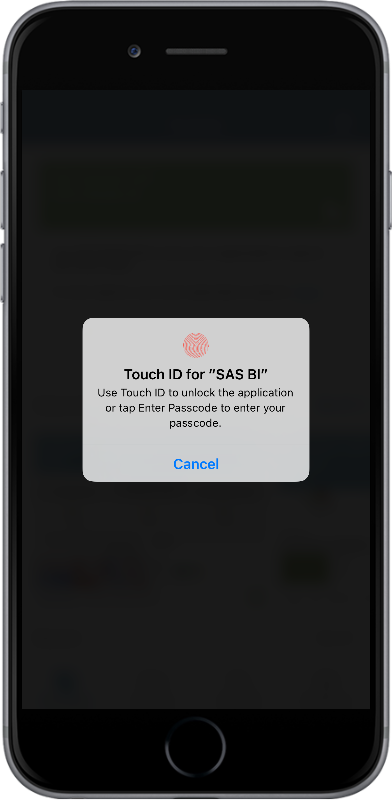The image features an iPhone with a Touch ID prompt displayed on the screen. The prompt reads: "Touch ID for SAS BI - Use Touch ID to unlock the application or enter your passcode." Below this message, there are two options: "Cancel" at the bottom and the option to "Enter Passcode," which is implied as part of the instruction, encouraging the user to authenticate by placing their fingerprint on the home button. The Touch ID icon, represented by a fingerprint, is prominently displayed above the text. The device appears to be requesting user authentication for accessing an application named SAS BI. The screenshot captures the entire phone, although the specific iPhone model is indeterminate. Visible elements include the home button at the bottom and the side buttons on the phone's edges. The background is minimal, focusing solely on the phone and the Touch ID prompt, with no other visible distractions.